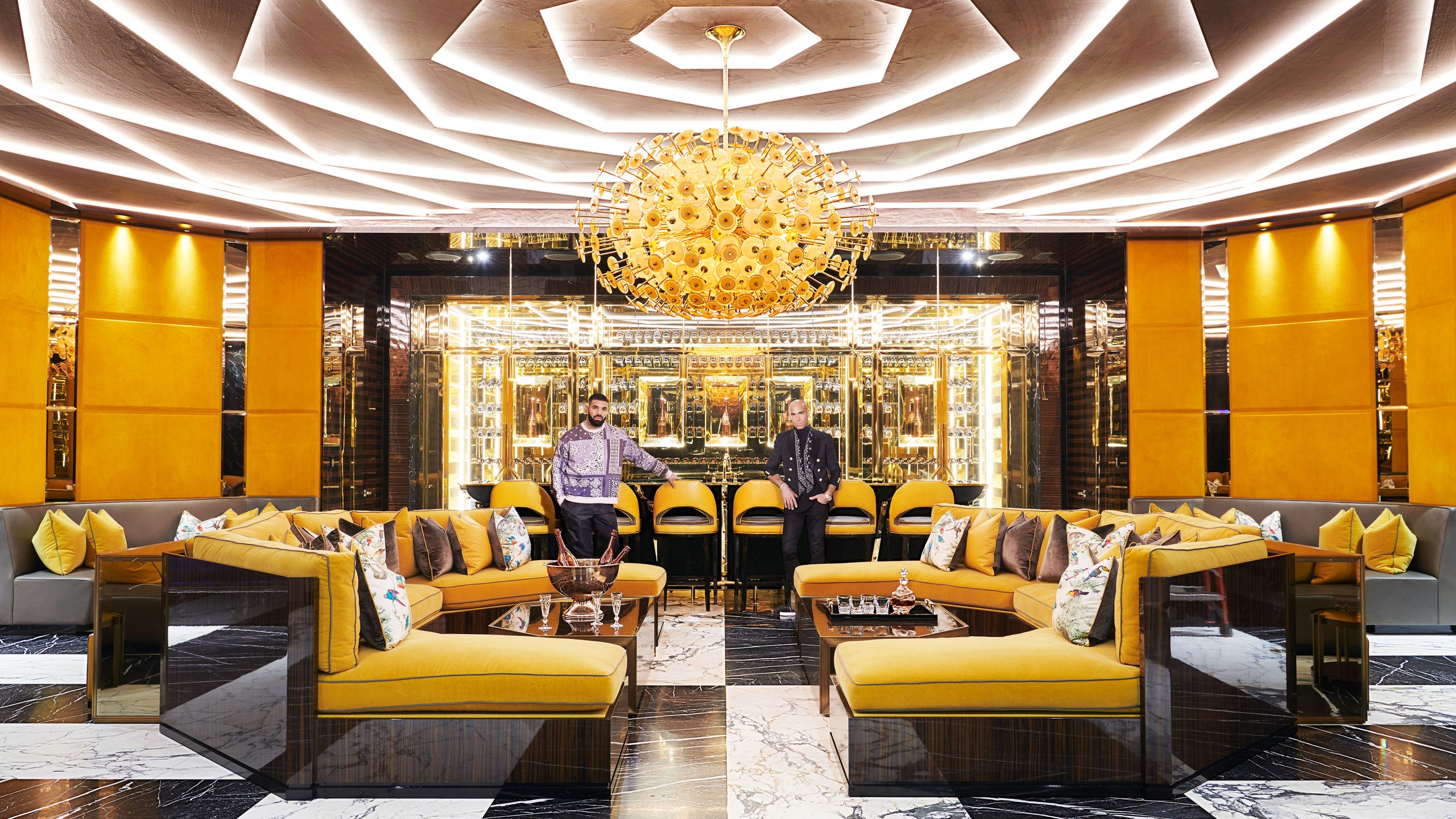This is a wide-angle photograph of a lavish, maize-yellow-themed lounge or lobby area, possibly a fancy clubhouse or hotel. The room features extensive yellow décor, including large, cushioned yellow couches with black marble bases arranged in semicircles, capable of seating around 15-20 people and adorned with several pillows. The floor has a striking black and white checkered marble pattern. Dominating the back of the room is a sleek bar area with six yellow chairs, lined with bottles on either side, including champagne and whiskey decanters with glasses arranged neatly.

The ceiling is an architectural masterpiece, featuring skylighting panels that allow natural light to pour in, illuminating the space. An abstract symmetrical design covers the ceiling, accentuated by a dramatic chandelier resembling an exploding yellow flower or peacock feather, adding to the room's opulence.

Two men stand in the foreground, to the slight left and right of the image's center. One, dressed entirely in black and bald, has his hands in his pockets, while the other, with black hair and a beard, wears black pants and a purple shirt, resting a hand on a chair. They appear to be gazing directly at the viewer, adding a touch of intrigue to the already captivating scene.